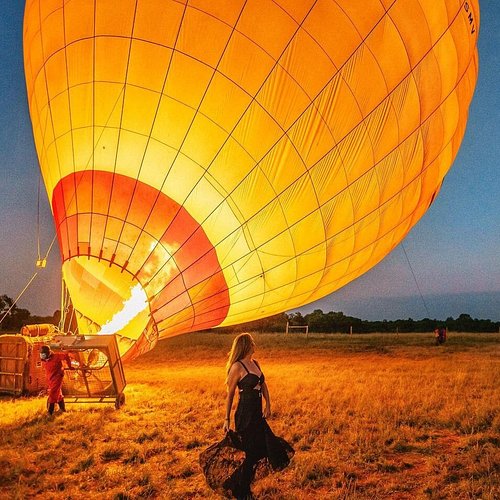In this color photograph taken at dusk, the setting sun casts a mixture of pink and orange hues across the sky, making the scene rich with warm tones. The image is slightly taller than it is wide and captures a woman in a long, black strap dress positioned at the bottom center of the photograph, her long brown hair cascading as she turns her head away, leaving her face unseen. She appears to either be standing or dancing gracefully, with her attention drawn towards a massive hot air balloon.

The hot air balloon dominates the central portion of the image, extending from the middle to the top edge, its vibrant yellow and reddish-orange sections emphasized by a network of black lines forming a patchwork of squares. The balloon, currently anchored to the ground with tether straps visible, is being inflated by a fiery flame shooting up from its base. The flame's glow illuminates the surrounding grassy field, which is more tan and brown in color, hinting at dead leaves and dirt.

Behind the woman, a man dressed in an orange outfit and white mask stands atop a wooden crate, handling a large fan used to fuel the balloon's fire. The scene is framed by a distant tree line of green foliage, stretching across the horizon beneath a deepening blue sky, creating a stunning backdrop to this captivating moment of a hot air balloon being prepared for flight.